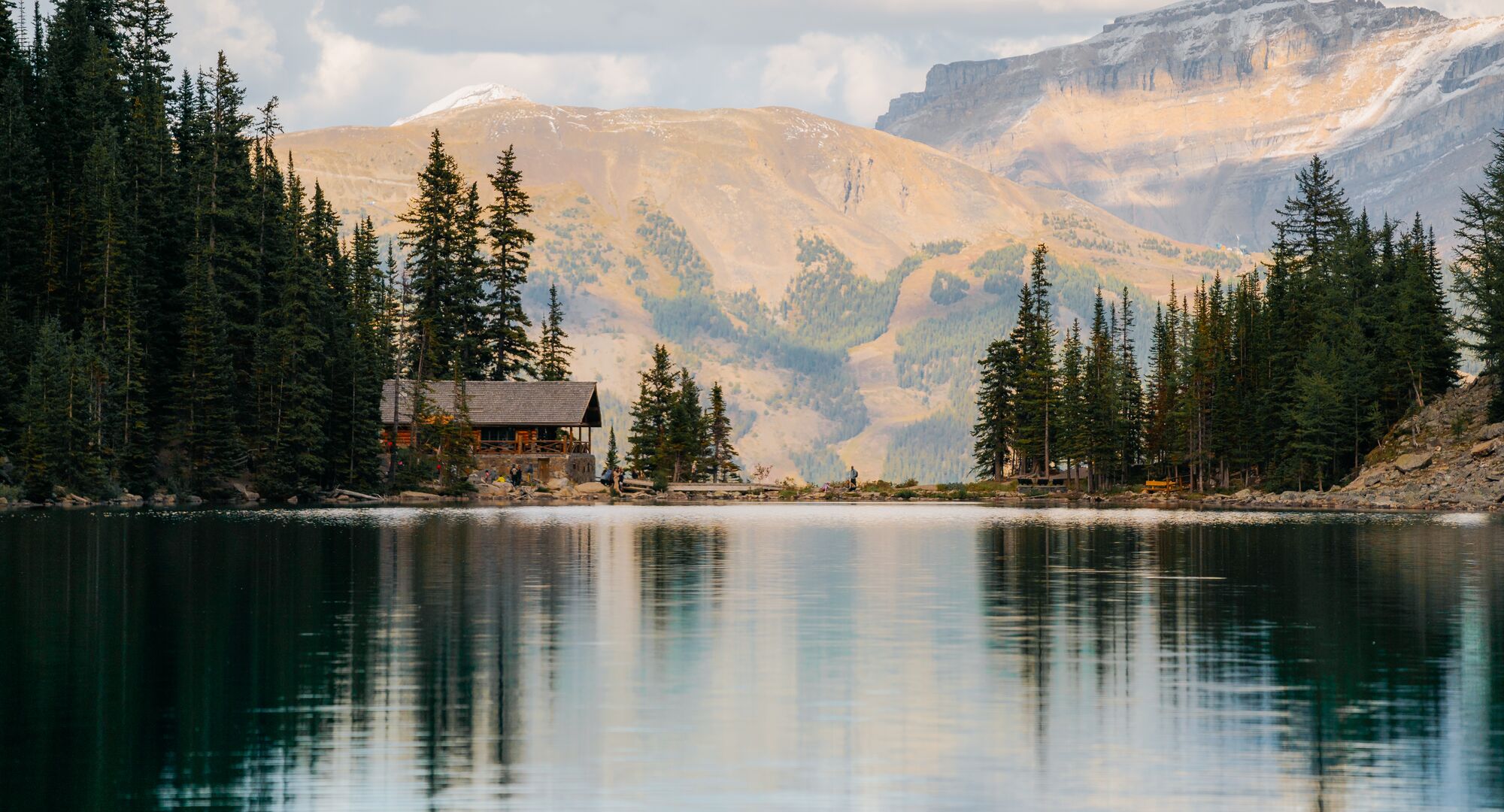This image captures a serene and expansive lakeside view framed by towering mountains in the background. The calm lake reflects the surrounding scenery, including dense tree coverage on both sides of the bank, though some ripples in the water are visible, particularly brighter in the center. On the left and right banks, evergreen trees stand in thick clusters, further adding to the natural beauty of the scene.

To the right, a rocky hill leads up to a wooded area, where a picnic table sits in front of some trees. A perceptible open section reveals a man standing at the lake's edge. On the left, there's an open structure with walls and a roof, possibly a pavilion or boathouse, featuring more picnic tables inside it.

In the distance, nestled among the trees, there appears to be a house or cabin, though the low resolution makes it difficult to discern its exact nature. This structure, built with wood and possibly housing boats, stands out with a thatched roof. Stretching higher, the mountainous background showcases varying levels of greenery and brush, with a hint of whiteness at the peaks, suggesting possible snow. The cloudy gray sky hangs over this tranquil, picturesque scene, adding a mild, reflective atmosphere.